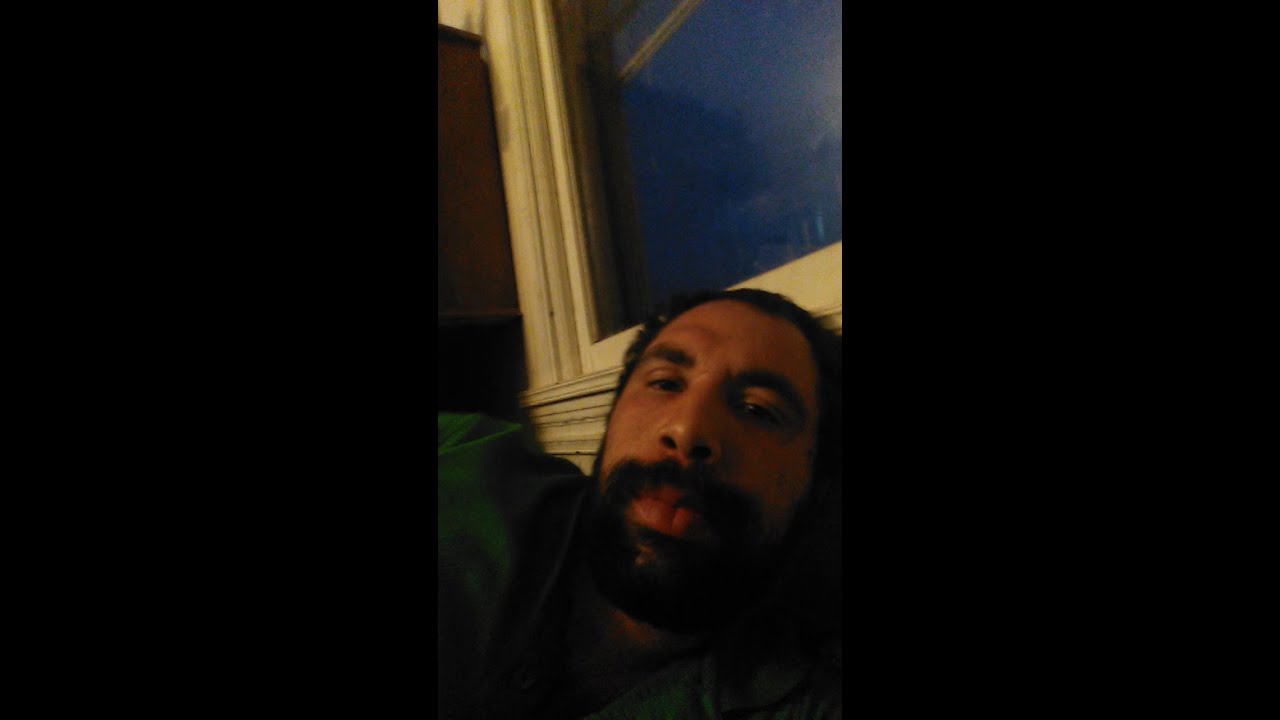In the image, a man of Middle Eastern or Hispanic descent rests his head against an old white window pane. His dark skin contrasts with his black beard and mustache, and his short black hair frames his face. He appears tired, with eyes that seem ready to close, suggesting he might be on the verge of sleep. Clad in a green shirt or jacket, he leans against the window, giving the impression of having either just been woken up or about to nod off. The nighttime sky outside the window is a deep blue, enveloping the scene in darkness, while the interior shadows create a calm, enclosed atmosphere. The photograph, likely a tall, narrow selfie, captures the man's serene yet weary expression, with larger black rectangles framing both sides of the image.